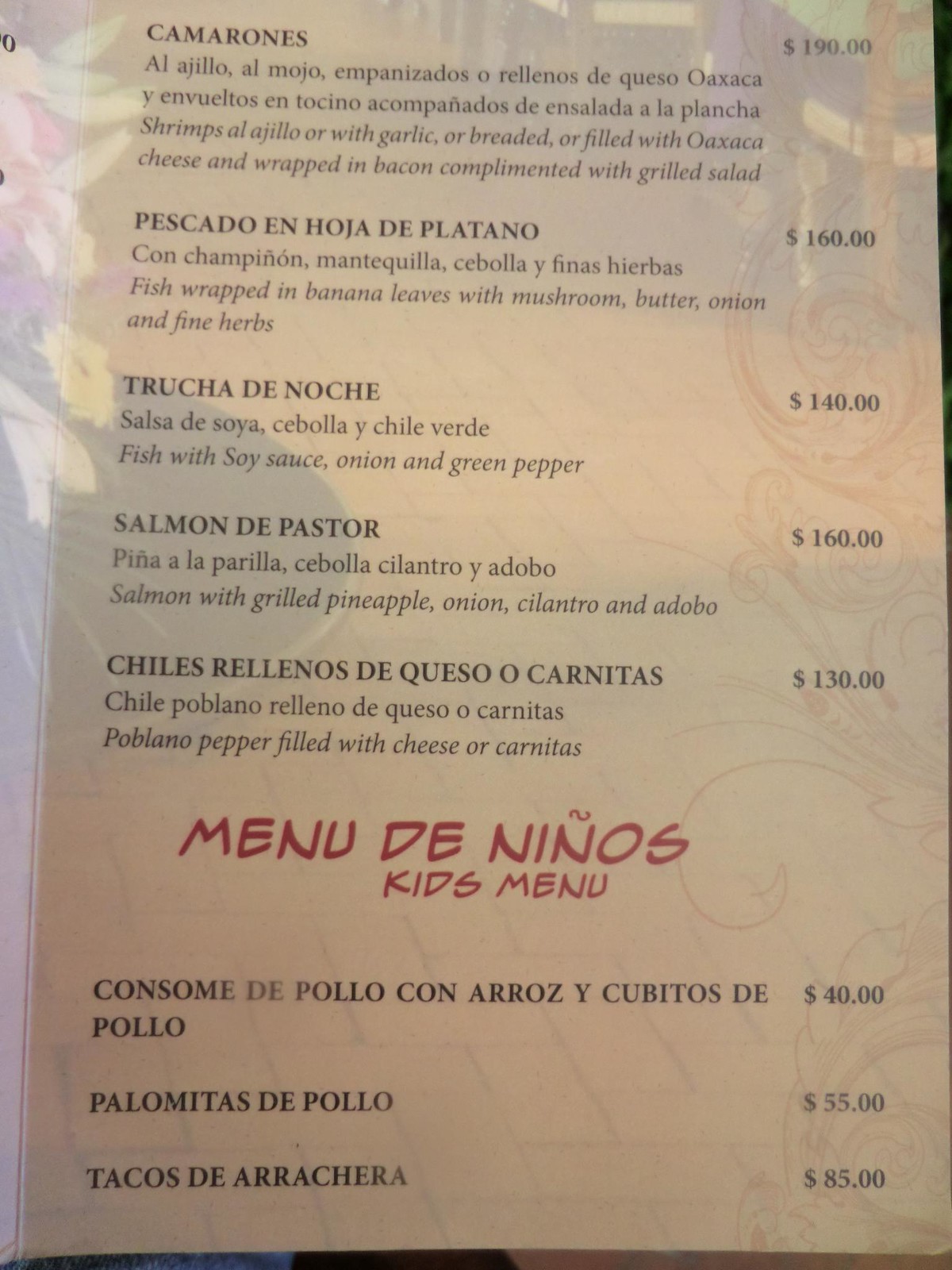The image displays a menu page presented on artistically designed yellow paper. The menu is bilingual, featuring items in both English and Spanish. At the top of the menu, the first item listed is "Shrimps with garlic or breaded or filled with Oaxaca cheese and wrapped in bacon, complemented with a grilled salad." Following this, the next entry is "Fish wrapped in banana leaves with mushrooms, butter, onion, and fine herbs," priced at $160. Next on the list is "Fish with soy sauce, onion, and green pepper," available for $140. Lastly, the menu features "Salmon with grilled pineapple, onion, cilantro, and adobo," which is offered at $160.